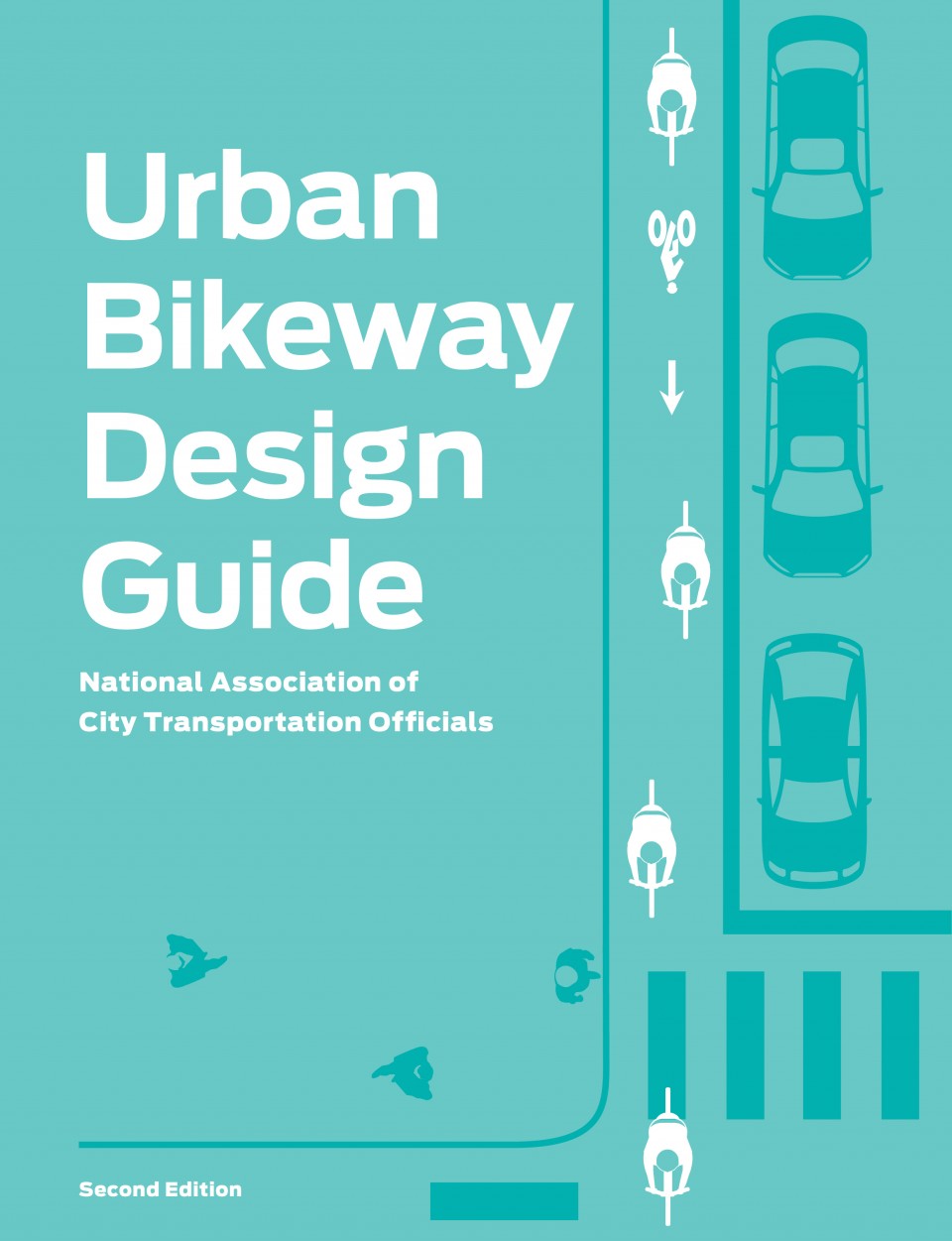The image is the cover of a textbook titled "Urban Bikeway Design Guide" by the National Association of City Transportation Officials, indicated in white text on the upper left. Also, in the lower left corner, in smaller white print, it says "Second Edition." The background is a blend of light turquoise and teal with various green and white shapes and illustrations. The central design features an artistic and somewhat vague aerial view of people riding bicycles, depicted as green figures leaning forward on handlebars. Along the bottom left, dark green pedestrian figures are crossing a road, while to the right, lighter-colored images show three vehicles driving downward. The overall style of the cover is artistic and abstract, focusing on urban transportation elements.